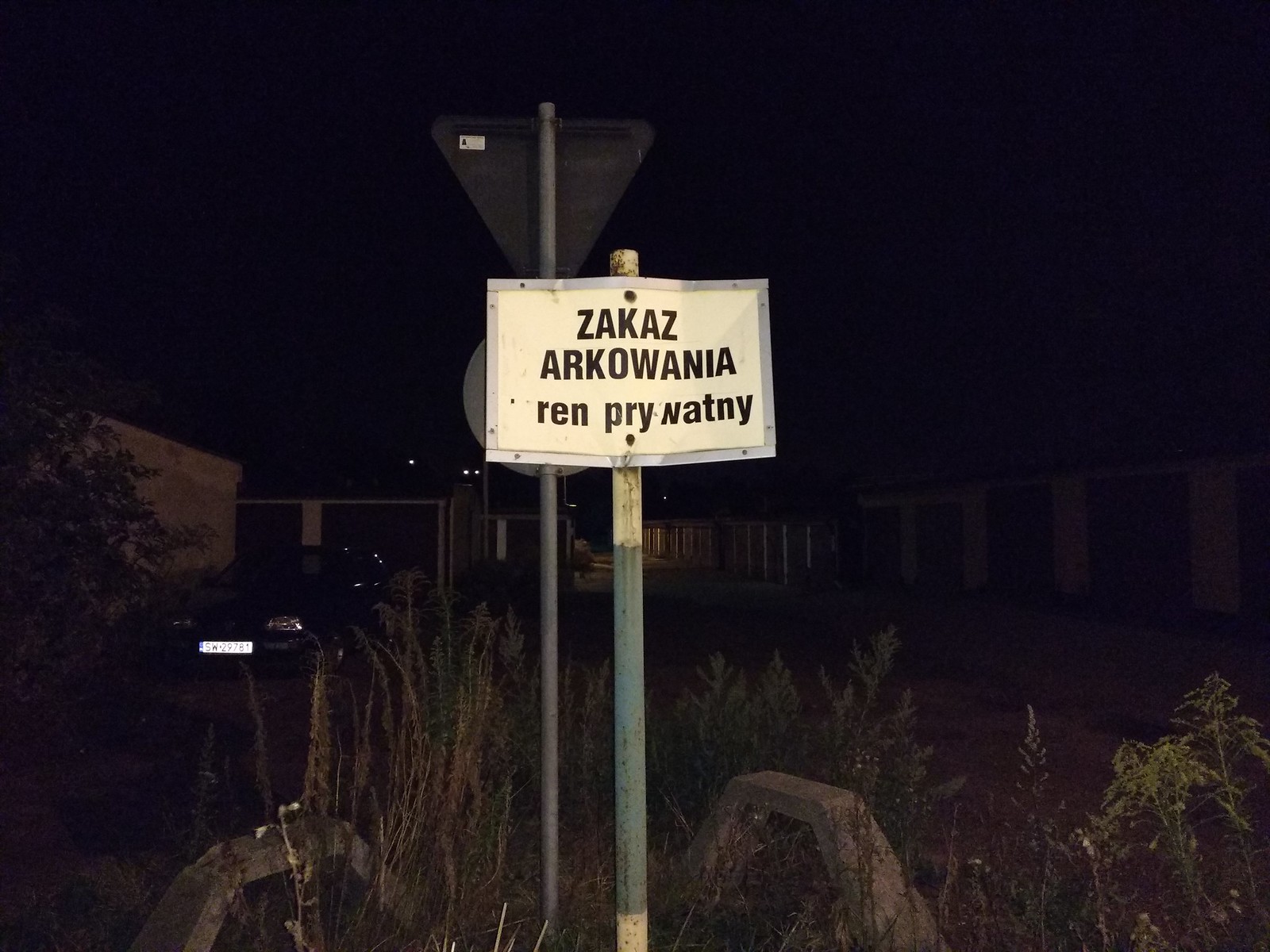This nighttime photograph captures a somewhat foreboding scene featuring a weathered yellow sign with black text, prominently displaying the words "Zarkav Arakawania" or similar, though the exact meaning is unclear. The sign is mounted on a wooden stick and framed by a silver boundary, appearing bent and unsteady. It stands amidst an unkempt yard, possibly the back area of an apartment complex, as indicated by a line of garages on the right, a parked black car with the license plate "SW 29781" to the left, and sparse tufts of grass and weeds breaking through the ground. The sky is pitch-black, emphasizing the nocturnal setting, and there are additional signs on weathered poles in the background, one circular and another triangular, both facing away from the camera. The overall scenery, marked by concrete blocks and scattered vegetation, evinces an aura of neglect and slight intimidation.